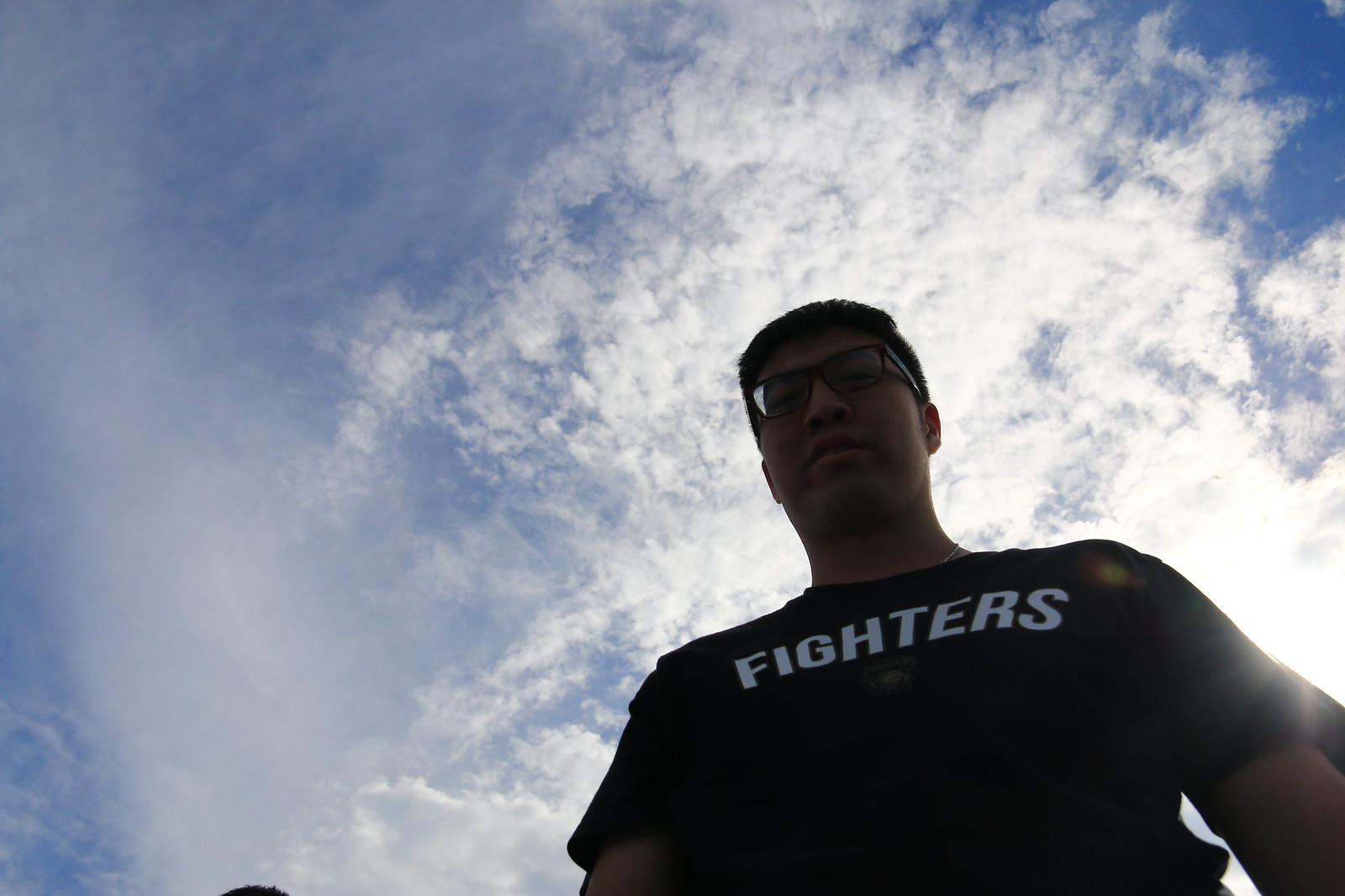The image is a selfie of a young man with short, dark hair and glasses, wearing a black t-shirt with the word "FIGHTERS" written in all capital white letters across the chest. The man is positioned slightly to the right edge of the image and is staring downwards. The background features a mostly cloudy sky with a sliver of blue visible and a sun flare towards the bottom right corner. Barely visible is the top of another person's head at the very bottom left of the image. No ground, buildings, or other elements are present in the background.